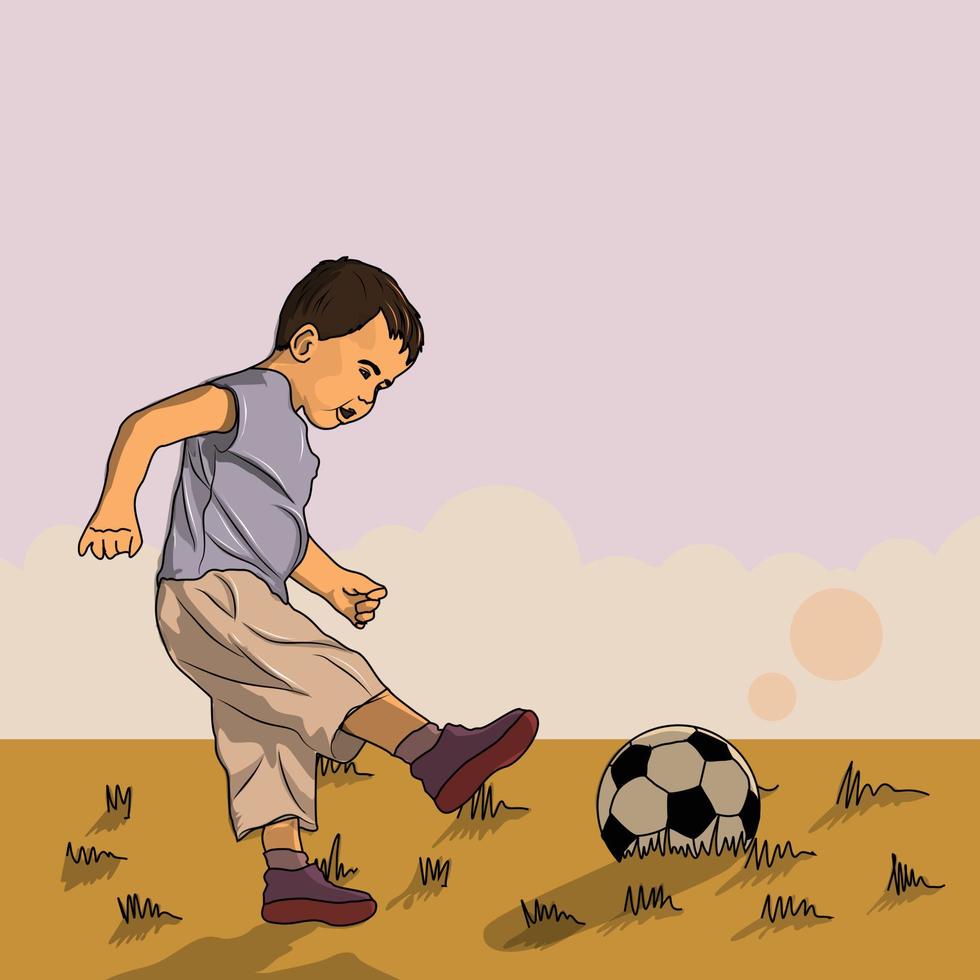This is a cartoon drawing of a young boy, seemingly around three to six years old, kicking a black and white soccer ball. The background starts off as a clear pink sky that transitions into a tan color halfway down, dotted with a few orange bubbles. The lower part of the backdrop displays a faded greenish-brown field, suggestive of dry grass, with darker greenish-brown squiggles representing individual grass blades. The boy, with brown hair, is dressed in a light blue shirt and ankle-exposing, ambiguous grey pants that seem neither fully shorts nor trousers. He sports white ankle socks and purple shoes with red bottoms. His expression isn't detailed, but he appears to be happy as he kicks the soccer ball, which casts a shadow on the ground. The scene suggests a sunny day, possibly in summer, due to the dry appearance of the grass and the boy's light clothing.